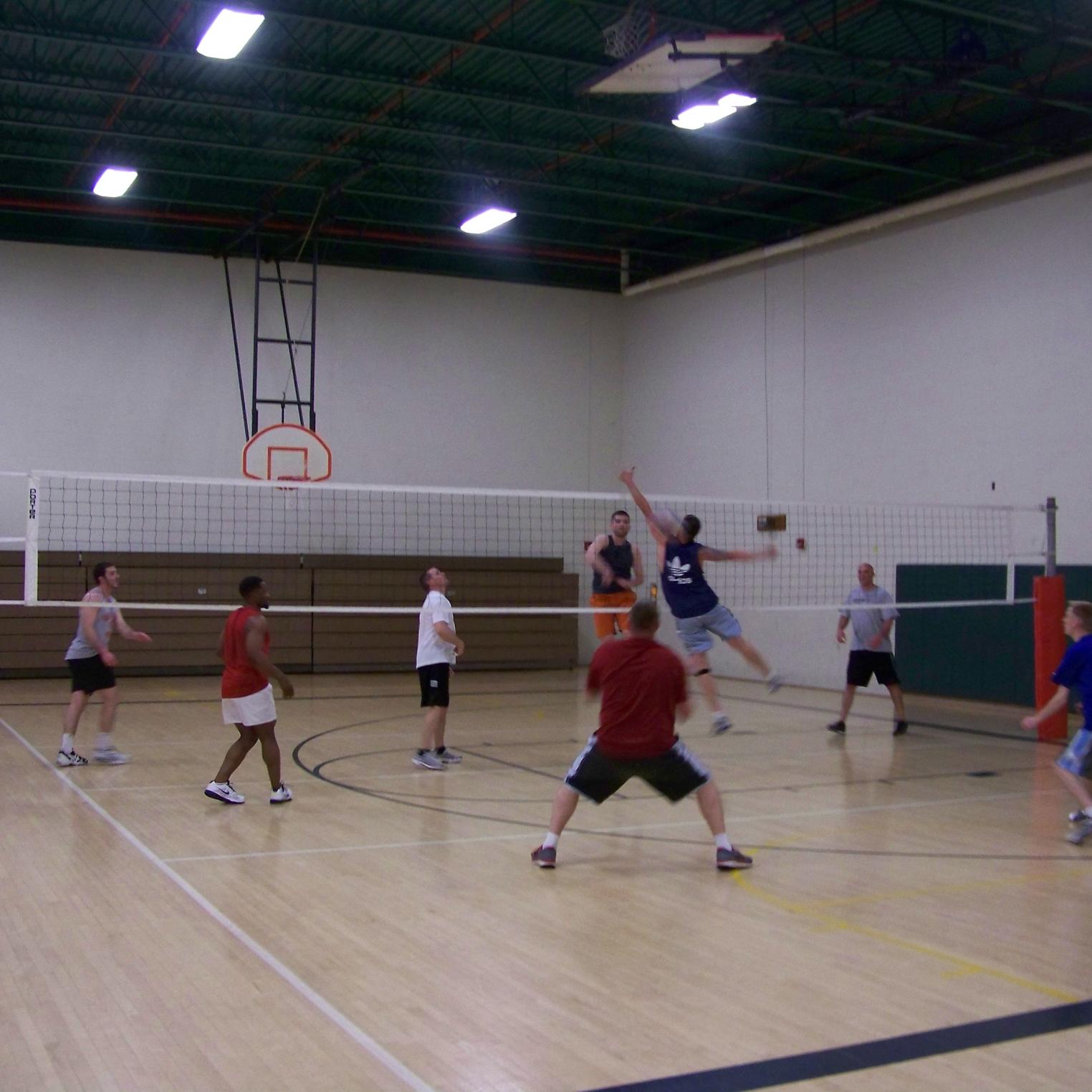This detailed color photograph, possibly a video freeze-frame, captures an intense moment in a men's volleyball game set inside a gymnasium. The match is being played on a multi-use court, clearly marked for basketball with visible etchings and a basketball hoop fixed high on the far wall. The gymnasium's bleachers are retracted against the wall, leaving ample space for the players.

The focus of the image is the volleyball action involving several players, primarily centered around a man in orange shorts on the far side who appears to have just hit the ball. A defender on the near side, dressed in a black Adidas shirt and blue shorts, is captured mid-air, seemingly attempting to block the shot. This dramatic leap near the net draws the viewer's attention, although the volleyball itself is mysteriously absent from view, suggesting it may have been obscured or is moving too fast to be captured. 

Surrounding these key players, several other men can be seen, some standing with their backs to the camera and others positioned around the court, all intently watching the play unfold. The lighting from overhead lights lends a sharp, realistic quality to this photograph, underscoring the immediacy and energy of the ongoing match.